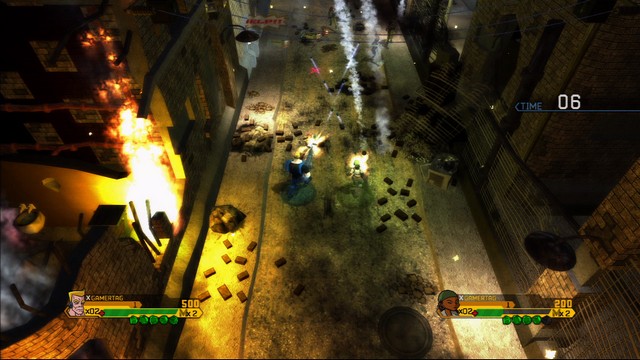The image is an in-game screenshot of a cooperative, two-player mobile shooting game, captured from a top-down perspective. The scene is set in a street flanked by buildings, with visible health and character bars on the left and right sides of the screen. Each player has a score indicator along with green icons likely representing lives; for example, one character with blonde hair has a score of 500 and 02 lives remaining, while a girl in a green hat has a score of 200 with the same lives remaining. The backdrop of the action includes a fire and explosions near the buildings on the left, creating an atmosphere filled with smoke. The players, positioned in the center, are firing northward at unseen targets. A timer reading "06" is displayed on the right side. The ground under the action features a table-like structure dotted with small brown objects and circular puffed shapes, illuminated by a bright yellow light that suggests an indoor scene but also compatible with the outdoor street setting.